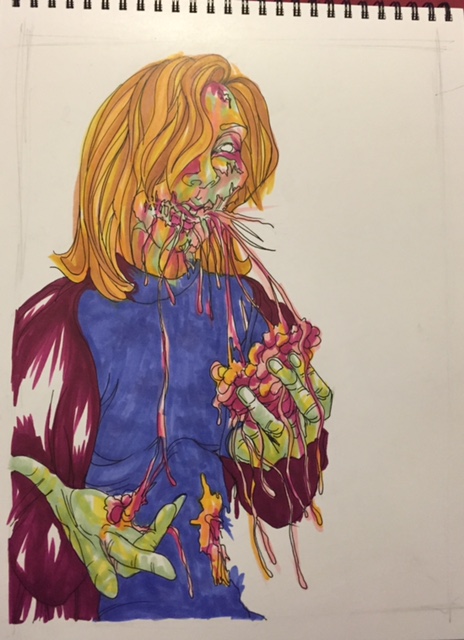A hand-drawn image in vibrant colored markers is depicted on the white or off-white pages of a ring-bound notebook, fastened by black rings through punched holes at the top of the booklet. The notebook is set against a red background that peeks through in the upper right corner. The drawing features a fantastical zombie-like creature with long blonde hair. The creature's face is a complex blend of greens, reds, oranges, whites, and possible hints of yellow hues, contributing to its eerie appearance. The figure appears to be ravenously consuming something red, with red and pink organic material spewing from its mouth. The creature’s hands are green and it is dressed in a purple sweater layered over a blue shirt. Intriguingly, a faint pencil outline of a box can be glimpsed surrounding the zombie-like figure, adding a subtle framing element to the artwork.